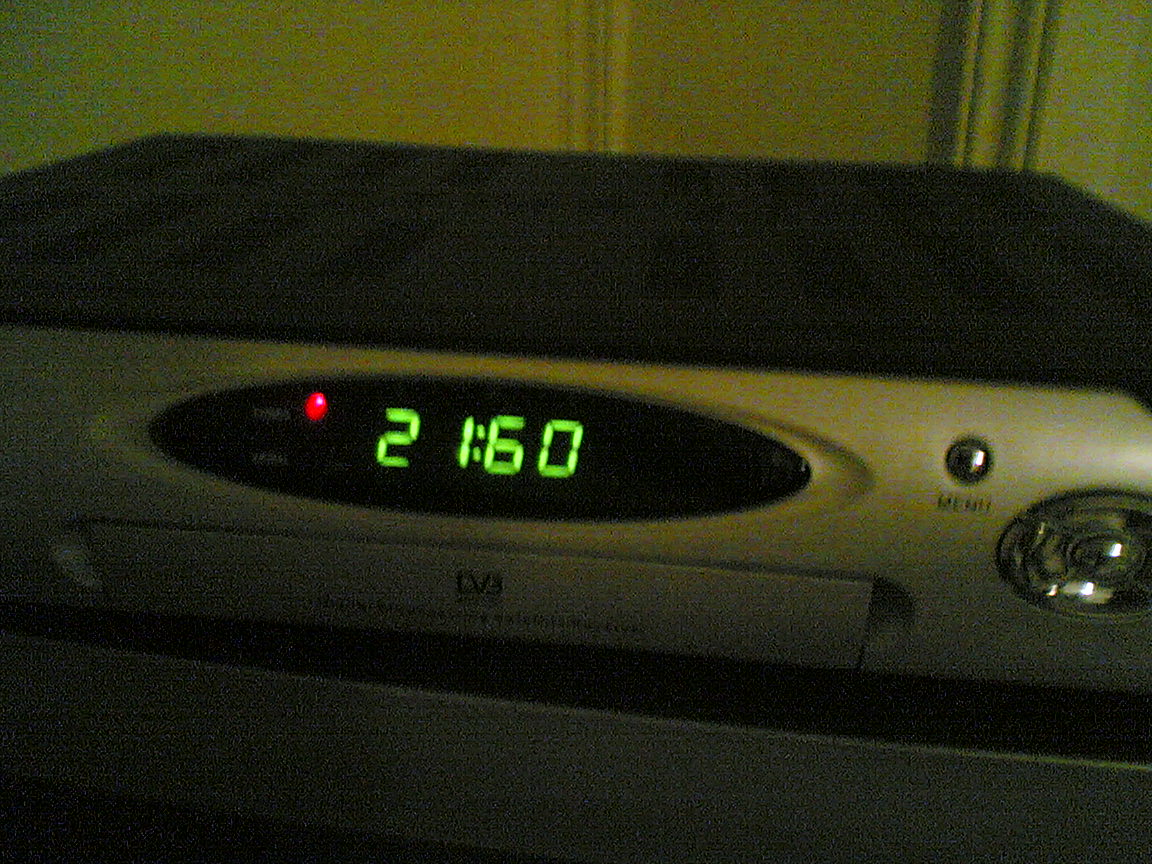This vintage-style color photograph captures a grainy, slightly blurry DVD player, evoking a nostalgic feel reminiscent of the 80s or 90s. The image, dimly lit, highlights the DVD player's front panel that has a black casing. Prominently displayed is an elliptical-shaped screen showing lime green numbers reading "21:60." To the right of this display are a series of controls, including a small silver circle marked "menu" and an array of directional buttons just off the frame. The power indicator, a small red dot, is lit up on the left side of the device. At the bottom, the DVD tray is closed, distinguished by a rim around the square door and black text "D/3" that resembles a web link. The entire machine rests on a gray platform with a greenish backdrop visible behind it.